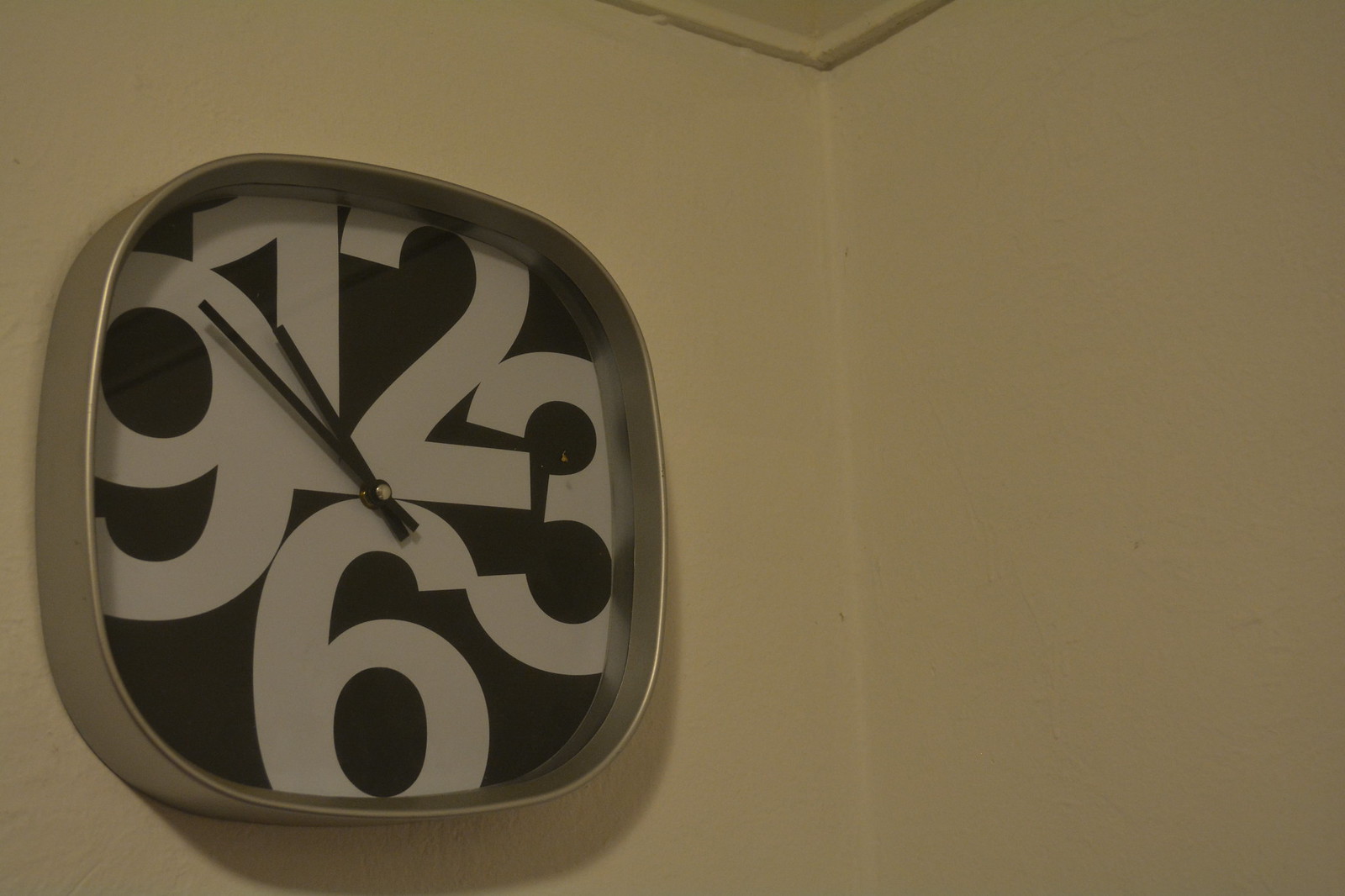This color photograph captures the corner of a room with pristine white walls. Mounted on the left wall is a prominent, modern clock featuring a square face encased in sleek silver metal. The clock's face is a stark black, contrasting with its large, bold white numbers, which are limited to 12, 3, 6, and 9. The current time displayed is approximately 9:50, although the exact time is somewhat ambiguous due to the clock's design. The clock boasts black hands, which are anchored at the center with a round silver detail. Notably, there is a noticeable mark or smudge near the 3 o'clock position, raising the question of whether this dirt lies on the inner surface of the clock or on the exterior glass that protects the face. The photograph captures the minimalist aesthetic and subtle imperfections of the scene.